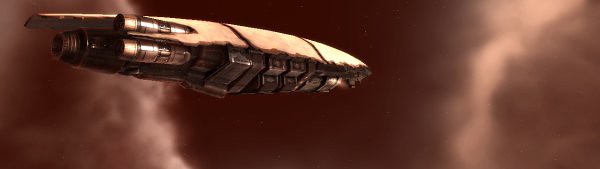The image resembles a still from a science fiction movie, depicting a sleek, bullet-shaped spaceship flying through space. The background is a captivating blend of dark bronze and white clouds. The spaceship's streamlined design features a distinctive turtle-shell-like top with three dividing lines, while the bottom showcases a square structure and visible engine components. At the rear, the spacecraft is equipped with one large, round jet propeller flanked by two smaller, similarly round propellers. There is also a noticeable hole on one side of the craft.